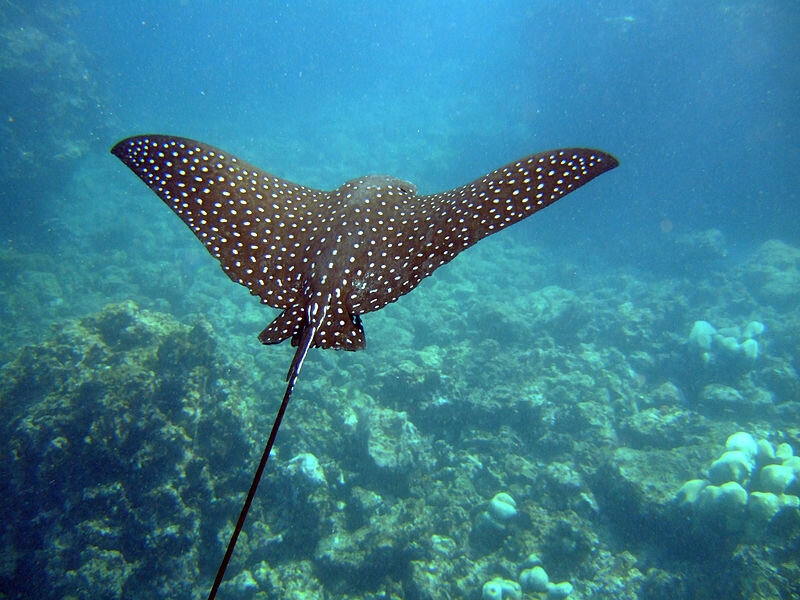The image depicts a stunning underwater scene, clearly illuminated by daylight with sunlight filtering through the water, which is a vivid, rich blue. The focal point is a stingray, which gracefully glides through the water, resembling a bird in mid-flight. The stingray, positioned in the middle to upper left of the image, has a dark, almost black or dark brown body adorned with distinctive white polka dots. Its wings are spread slightly at an upward angle, and its long tail with a barb extends straight behind it. The ocean floor below is somewhat dark and grayish, littered with various white seashells and dotted with rocks, some showing signs of moss or algae growth. The overall scene has a slightly hazy or foggy quality, enhancing the mystique of the underwater environment.